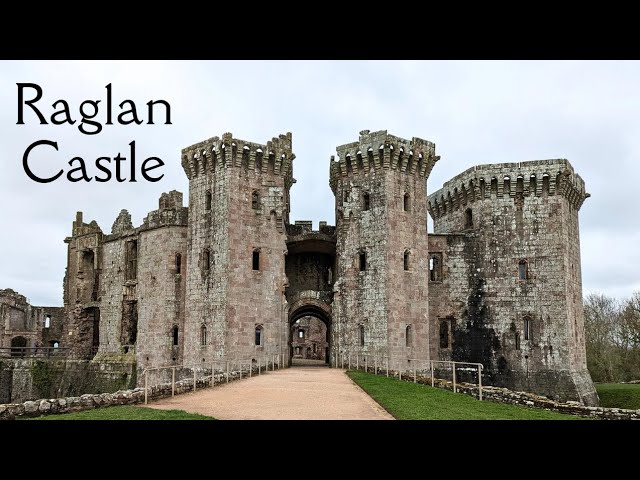In this photograph, the top and bottom portions feature a black border that frames the image. At the top, in bold black letters, the name "Raglan Castle" is prominently displayed. Against a charming backdrop of a clear, blue sky, the ancient stone structure of Raglan Castle stands resolute, surrounded by lush greenery and mature trees. The manicured lawns contribute to the picturesque setting, further encapsulated by a weathered stone fence that delineates the castle's perimeter.

Leading up to the castle’s main entrance is a concrete sidewalk, inviting visitors to explore its historical grandeur. The castle's venerable age is evident; the stones are faded and mottled with patches of white, whispering tales of centuries gone by. The structure comprises several square-topped buildings, each supported by protruding bars that help fortify their peaks. These buildings are interconnected by narrow walkways, providing a labyrinth of passageways that evoke medieval intrigue.

Dominating the façade is a formidable, large wooden door that serves as the main entrance, standing as a guardian to the secrets and stories of Raglan Castle.